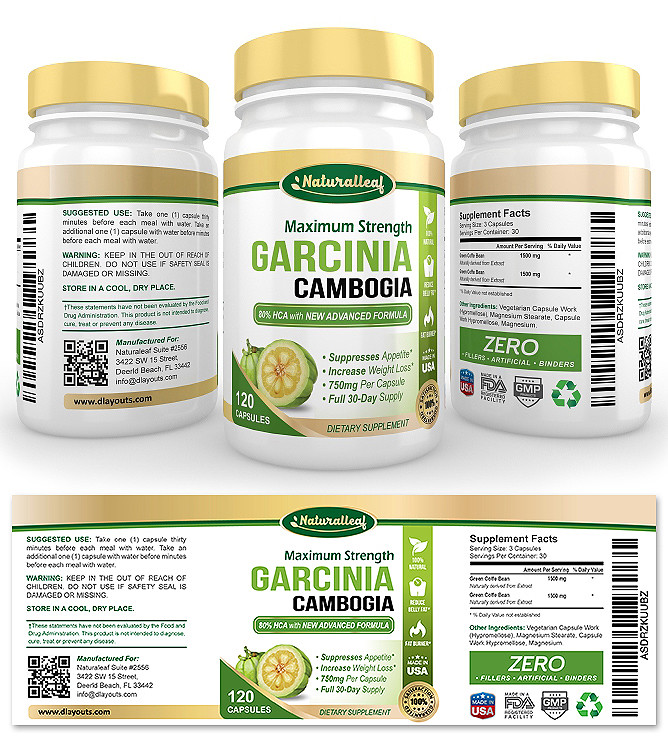The image shows three white pill bottles with gold screw caps, labeled as dietary supplements. Each bottle displays "Maximum Strength Garcinia Cambogia," made by a company called Natural Leaf. The green label with white and gold accents details the supplement's features: it contains 700 mg per capsule, offers a full 30-day supply, and includes 120 capsules in total. The front label highlights its appetite-suppressing and weight loss benefits. The middle bottle's label shows the product's name and main advertising points, while the other bottles provide the suggested use, warning labels, storage instructions, and Supplemental Facts. Additional information includes claims of zero fillers, artificial ingredients, or binders, and it references FDA information. A visible label beneath the bottles contains further details and a website, www.dlayouts.com, for more information on the product.